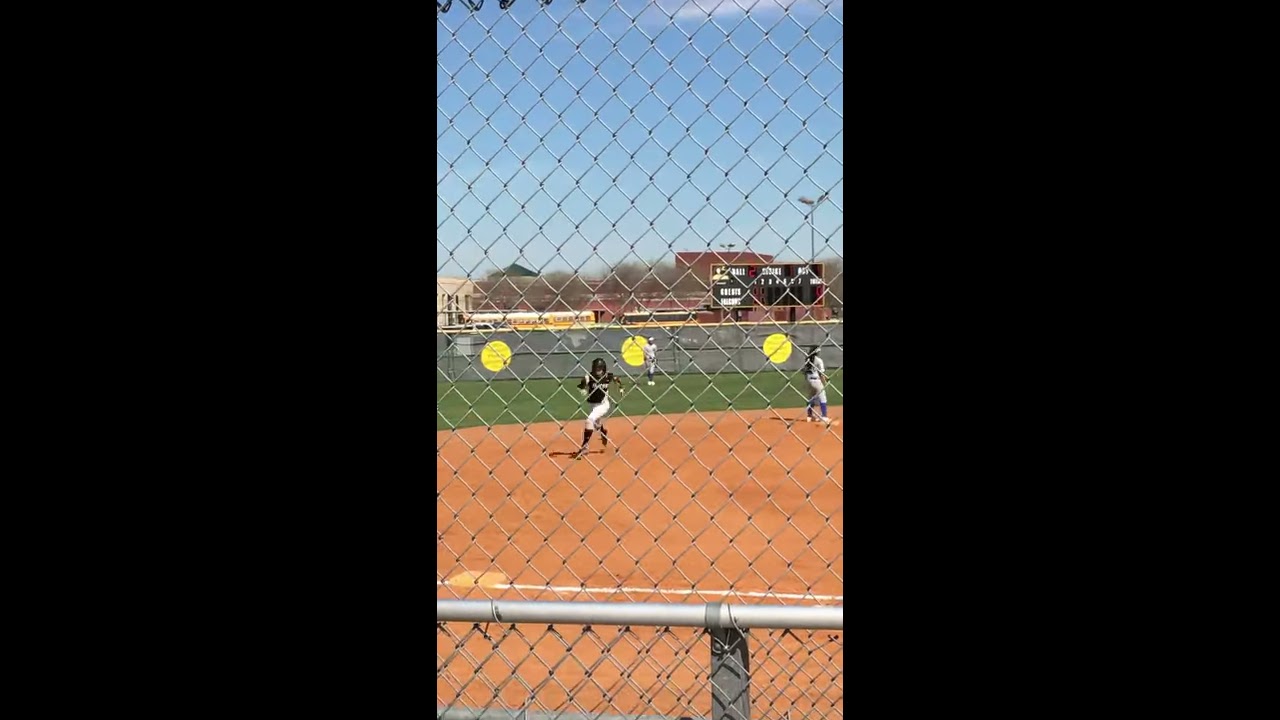This image is a color photograph taken in portrait orientation, possibly with a mobile phone, as it occupies a tall aspect ratio and is bordered by black on both the left and right sides, giving prominence to the central visual. Through a silver chain-link fence, the viewer can see a vivid scene of a baseball or softball field. The field has a reddish-brown dirt surface with white chalk lines and green grass in the distance. There are three players on the field, likely women, dressed in uniforms; one in white pants and a black top with a black cap appears to be running towards a base, and another player is observed in a white uniform. In the background, there is a somewhat blurry scoreboard and a few buildings, with a notable round structure and what could be a school bus. The scene is illuminated by tall structures resembling streetlights, contributing to the sense of a daytime sports event.